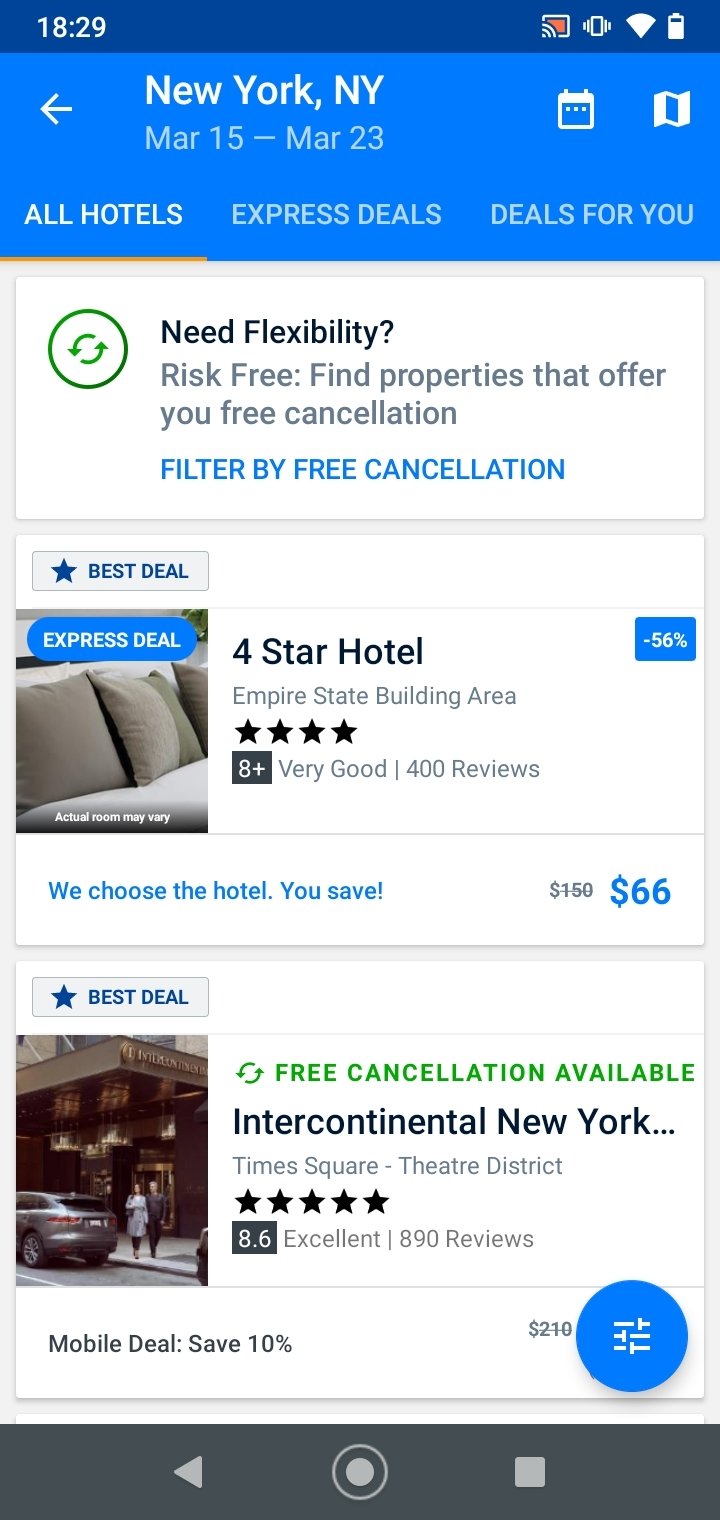This is a detailed description of a cropped screenshot from the Expedia mobile app. 

At the top of the image, there's a blue header displaying "New York, New York" in bold white letters. Immediately below it, the dates "March 15 to March 23" are indicated, accompanied by a small white calendar icon and a map icon to the right. 

The bottom of the header features categories like "All Hotels," "Express Deals," and "Deals for You," arranged horizontally.

The background beneath the header is white. At the top of this section, "Need Flexibility" is written in bold black letters. Underneath, in gray text, the message reads: "Risk-Free, find properties that offer you free cancellation." Following this, a call-to-action in bold blue font says, "Filter by Free Cancellation." To the right of "Need Flexibility," there's a green refresh icon.

Below this informational block, a list of search results begins. The first result features a gray bar labeled "Best Deal" with a blue star icon on the left. Directly beneath, there's a thumbnail photo of a bed, overlaid with a blue oval that reads "Express Deal" in white font.

To the right of the thumbnail, "Four Star Hotel" is prominently displayed in bold black letters, with "Empire State Building Area" noted below in small gray text. Underneath this, there are four colored-in black stars and a rating that says, "B-Plus Very Good." To the right, the review count "400 Reviews" is indicated. The bottom right corner of this result displays a price of "$66" in blue text, with a note to the left that says, "We Chose This Hotel, You Save."

Below this, the second result is briefly shown for the "Intercontinental New York Hotel."